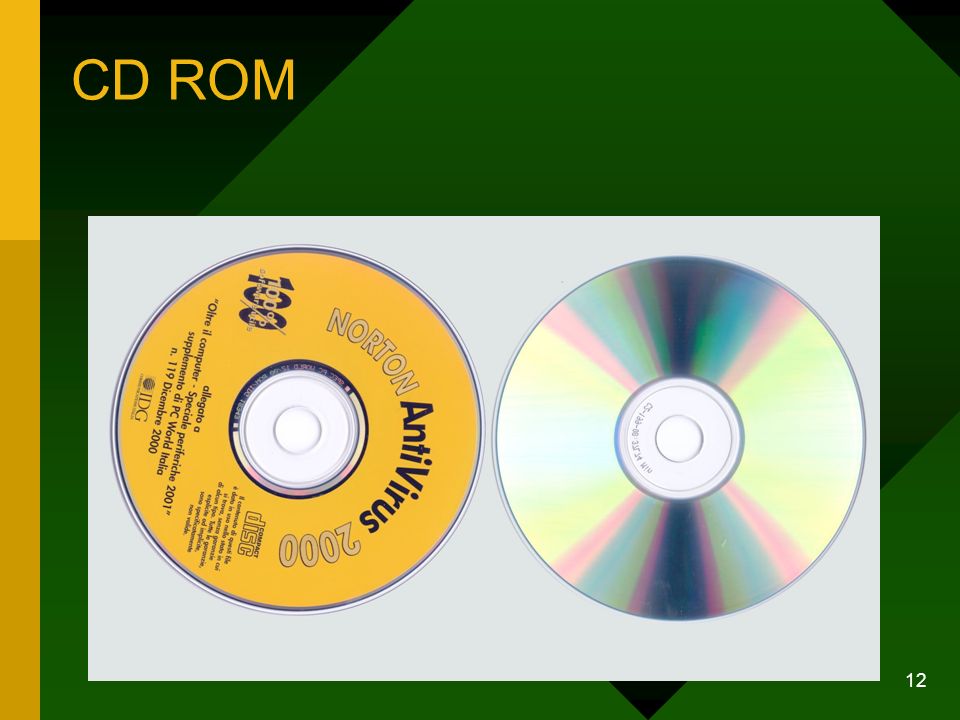The image features a detailed presentation of a CD-ROM. The upper left corner prominently displays the word "CD-ROM" in bold yellow text against a computer-generated green background featuring various shades and boxy lines. Centrally positioned within a white rectangle are two discs. The left disc displays the front of a CD-ROM, which is yellow and bears the title "Norton Antivirus 2000" along with black lettering and additional details that are difficult to read. To the right of it, the underside of the CD is shown, exhibiting a typical CD-ROM's translucent multicolored reflection. In the lower right corner of the image, the number "12" can be discerned, appearing in white text.